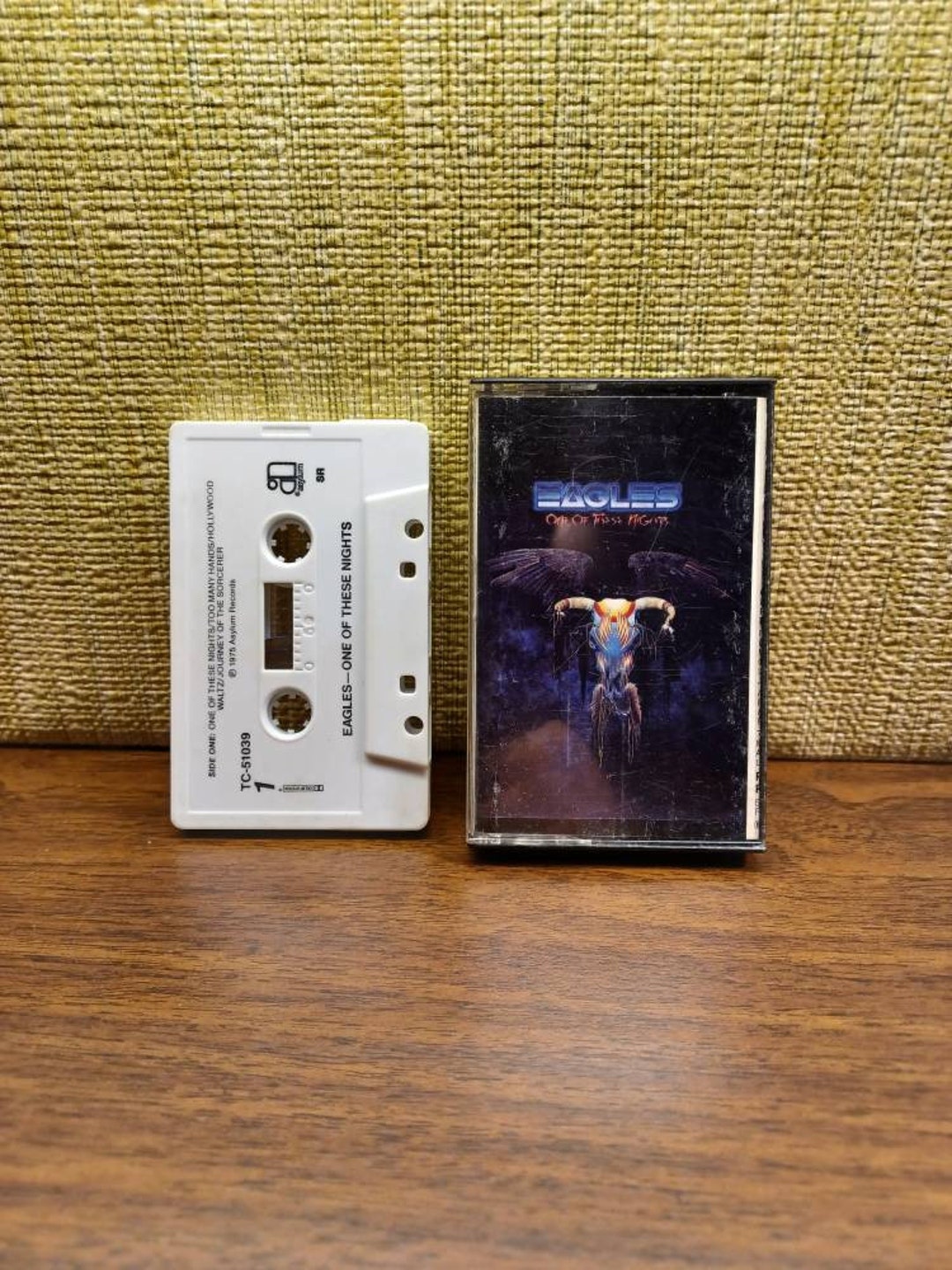The image showcases a vintage audio cassette tape and its case, both prominently featuring the band name "Eagles" and the title "One of These Nights." The white cassette tape, which displays two circular reels for rewinding, is positioned upright on its left side adjacent to the case. The cassette case, which is predominantly black, features intricate artwork—likely a depiction of a winged creature or an abstract design—alongside the band's name and album title. Both items rest on a wooden surface and lean against a tan and white woven wicker piece, possibly a basket or chair, enhancing the nostalgic and rustic setting.